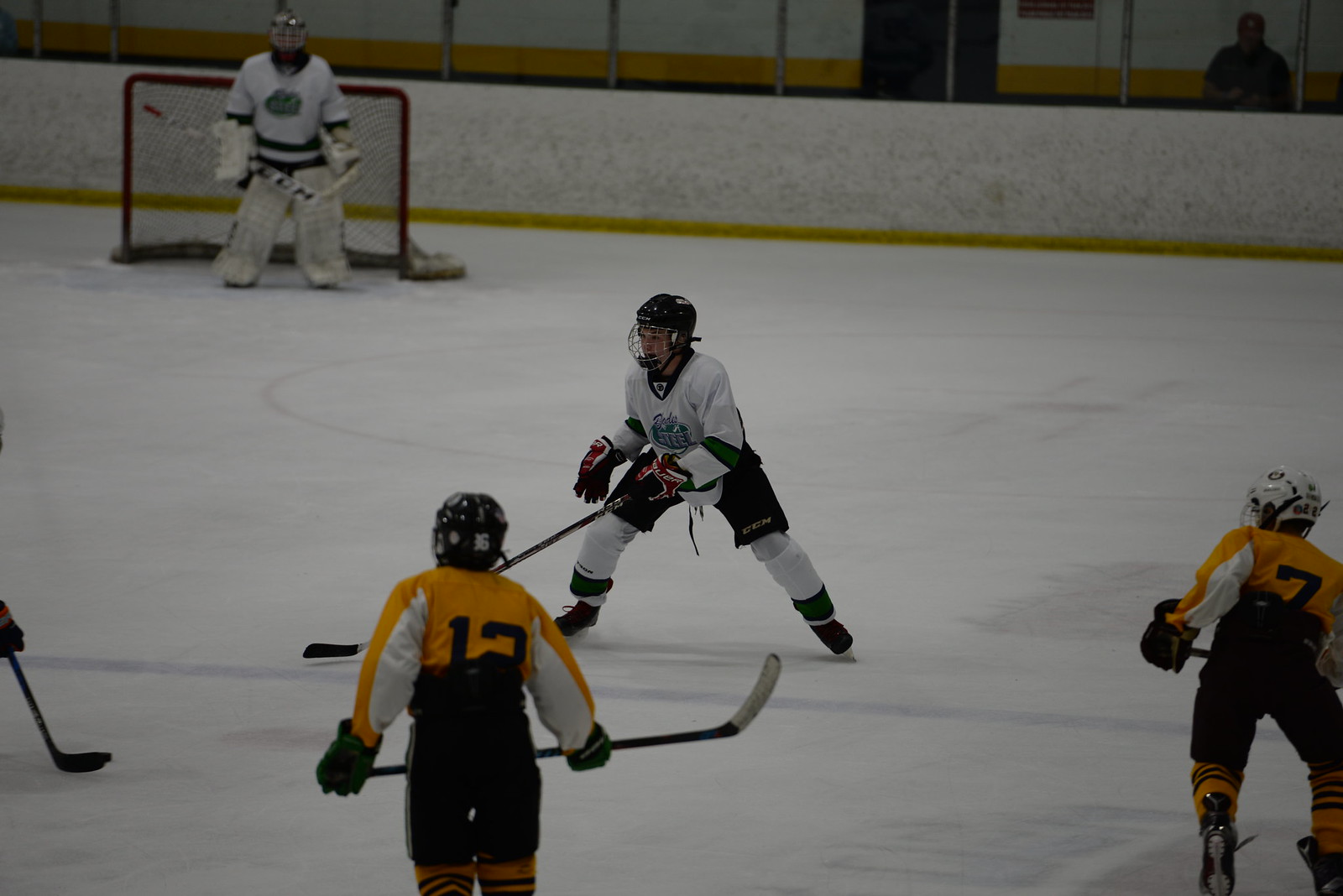This detailed indoor hockey game scene features several players on an icy surface, captured from an elevated vantage point. At the center of the image, multiple players in full gear are visible, including those in white jerseys with blue stripes and players in yellow and white uniforms. Focus is drawn to a white-jerseyed goalie standing by a red goalpost in the upper left corner, framed by the white wall and protective glass lining the rink. The goalie’s uniform features blue stripes and a distinctive logo. One player in a yellow jersey, marked with a partially visible number 12 or 13, has their back to the viewer, wearing a black helmet. Off to the right edge, another yellow-jerseyed player can be seen, also with their back turned. A lone spectator, seated in the bleachers, watches the game unfold. The image captures the dynamic pursuit of the puck amid the bright contrasting colors of the players' uniforms and the smooth, painted ice below them.